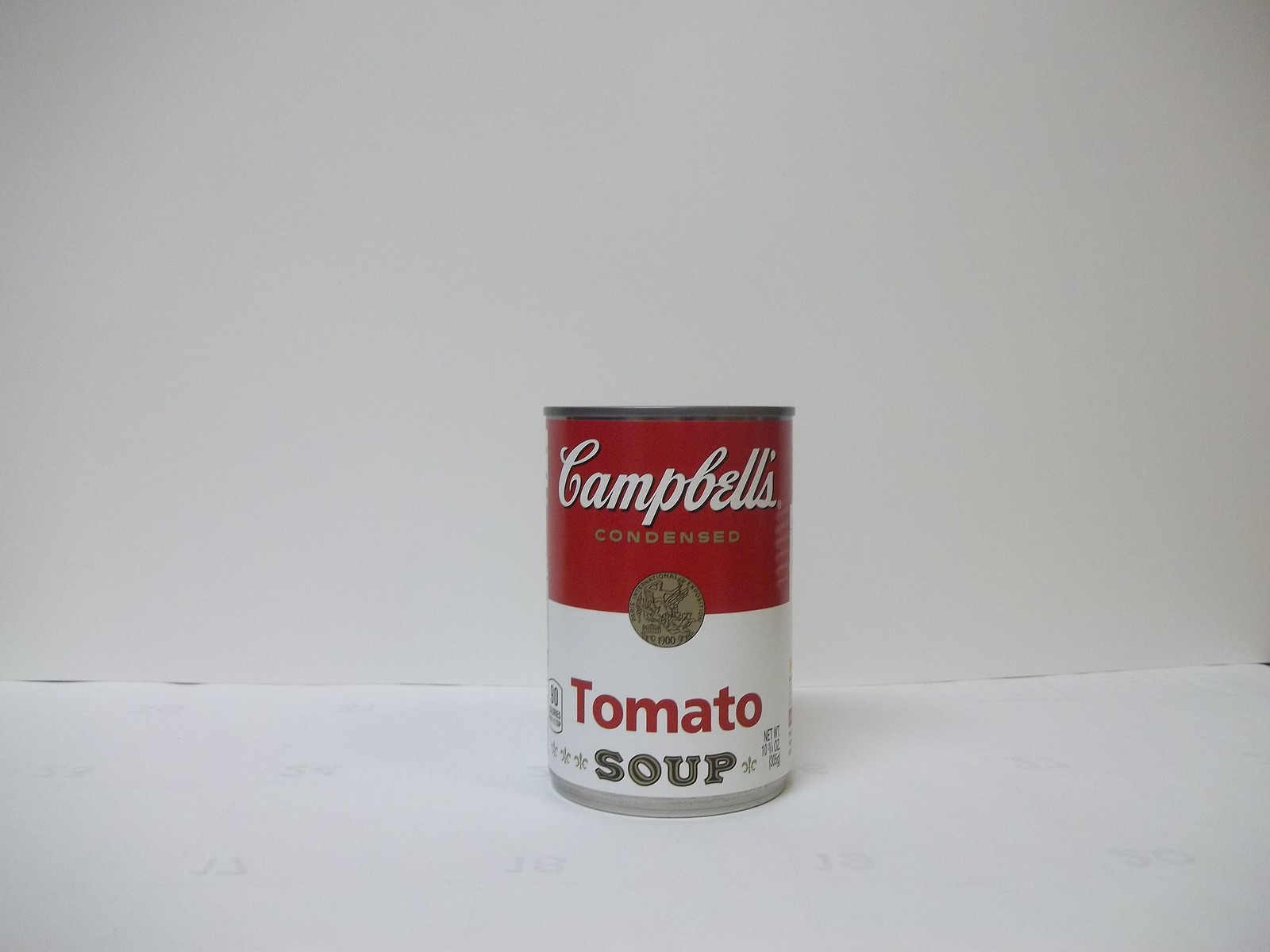This image features a 10.75-ounce can of Campbell's tomato soup, prominently displayed against a light gray background that appears white under certain lighting conditions. The can is positioned on a light gray surface, and it casts subtle shadows to the right and left. The can's label is typical of Campbell's soup: the top half is red and the bottom half is white. "Campbell's" is written in white cursive at the top, followed by the word "condensed" in gold text. A gold circular emblem resembling a coin is centered on the label, straddling the red and white sections. In the lower white section, "tomato" is written in red, and below it, "soup" is displayed in a blackish or grayish color, outlined in silver, flanked by a fleur-de-lis on each side. The can does not feature a pull tab, indicating that a can opener is necessary to open it.